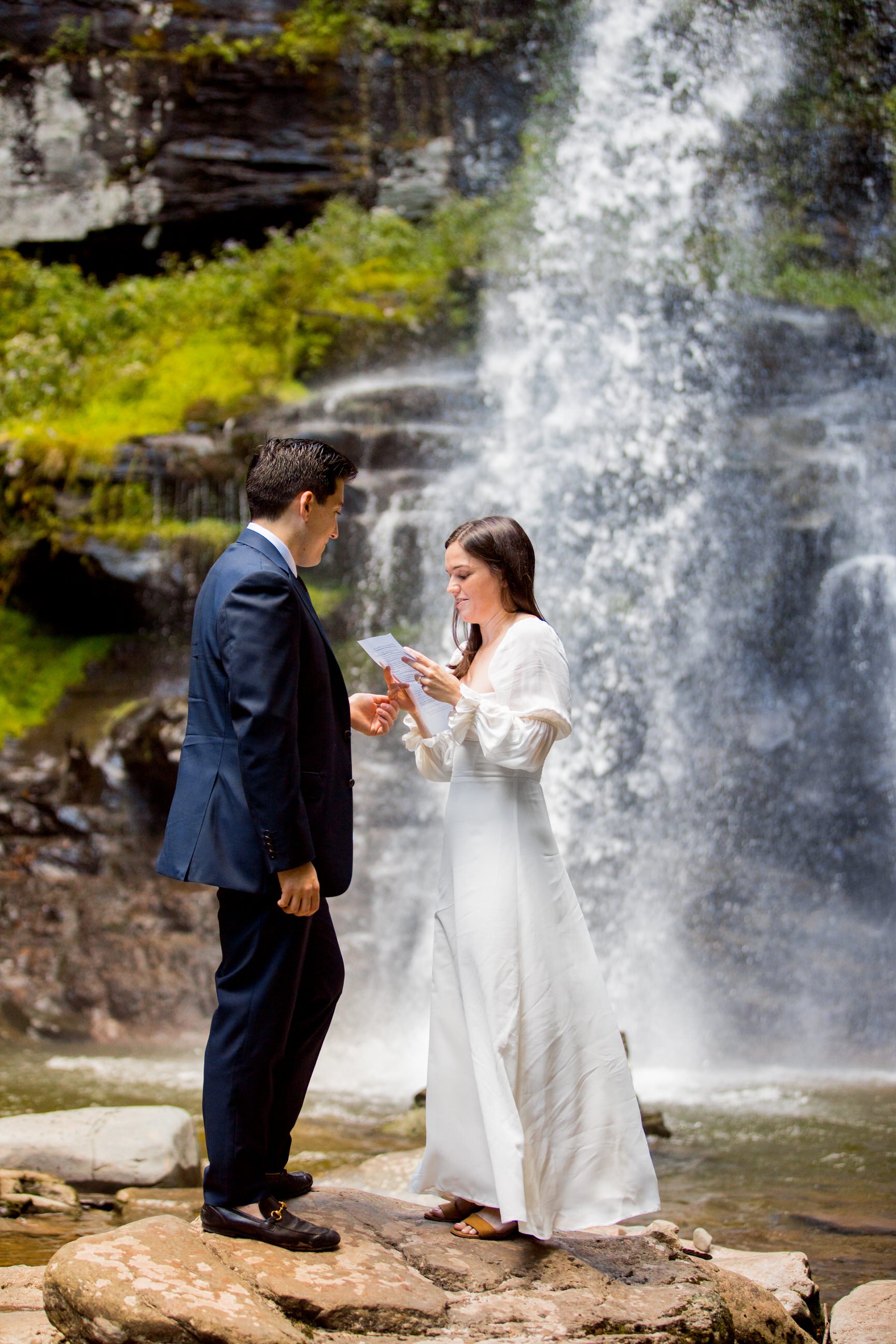In this captivating photograph, a well-dressed couple stands gracefully in front of a majestic waterfall set in a serene natural landscape. The man, clad in a dark blue suit with matching trousers and black loafers, gazes down with a smirk at the woman beside him. His jet-black hair adds to his polished appearance. The woman, adorned in a flowing white dress that resembles a wedding gown, holds a piece of paper with both hands, seemingly in the middle of reading aloud. Her elegant attire and the document suggest a moment of significance, possibly a vow or a heartfelt message. Behind them, the waterfall cascades down a rugged, mountainous terrain, surrounded by large rocks, lush grass, and diverse plant life. This idyllic scene is completed by the small body of water at the base of the waterfall, over which the couple stands on a prominent rock, adding to the romantic and picturesque quality of the image.